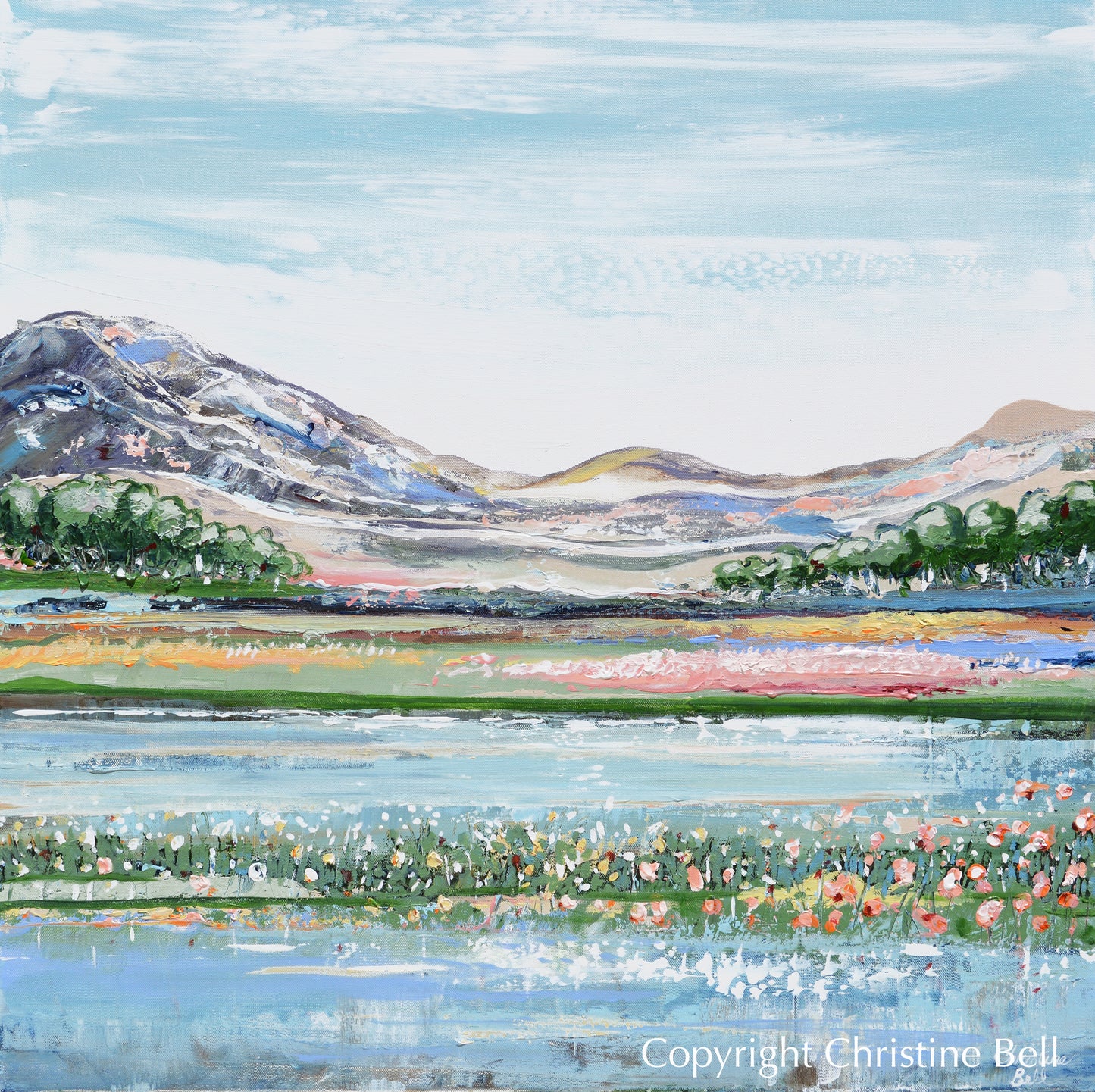The artwork is a square painting titled and signed "Copyright Christine Bell" in white letters at the bottom right-hand corner. The scene is a detailed portrait of a natural landscape set against a vibrant blue sky adorned with wispy, horizontal white clouds. Below the sky lies a range of visually striking mountains, primarily brown but interspersed with subtle hues of pink, blue, light red, and yellow to create a dynamic shadow effect. Flanking the mountains on either side are groups of large, green canopied trees with rounded tops and white bases. 

In front of the tree line stretches a meadow adorned with an array of colorful flowers in shades of pink, white, yellow, blue, and orange. The meadow transitions into a greenery-filled strip with more flowers and eventually leads to a light blue pond. Within the pond area, there appears to be patches of green grass dotted with flowers, further enhancing the idyllic and serene atmosphere of the painting. This composition creates a harmonious blend of wetlands, dry land, lush vegetation, and tranquil water, all culminating against the majestic backdrop of mountains and sky.